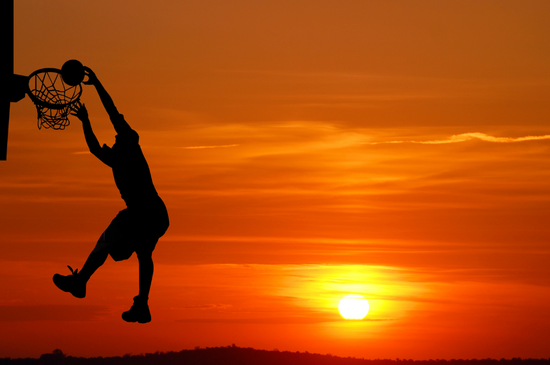The image portrays a stunning sunset scene at an outdoor basketball court, where the sun, a radiant yellow orb, sets over the horizon, casting the sky in vivid hues of yellow, orange, and golden tones. The upper part of the picture gradually darkens as the sun descends, reflecting its light beautifully on the water below. A basketball player, captured as a striking black silhouette, leaps into the air in a dynamic pose, dunking the ball into the hoop. The silhouette reveals the player's attire—shorts and tennis shoes, with discernible details like the tongue of the sneakers. The basketball hoop, net, and backboard stand clearly outlined against the colorful sky. The background shows a shadowy, tree-lined hill, completing this creative and atmospheric photograph.